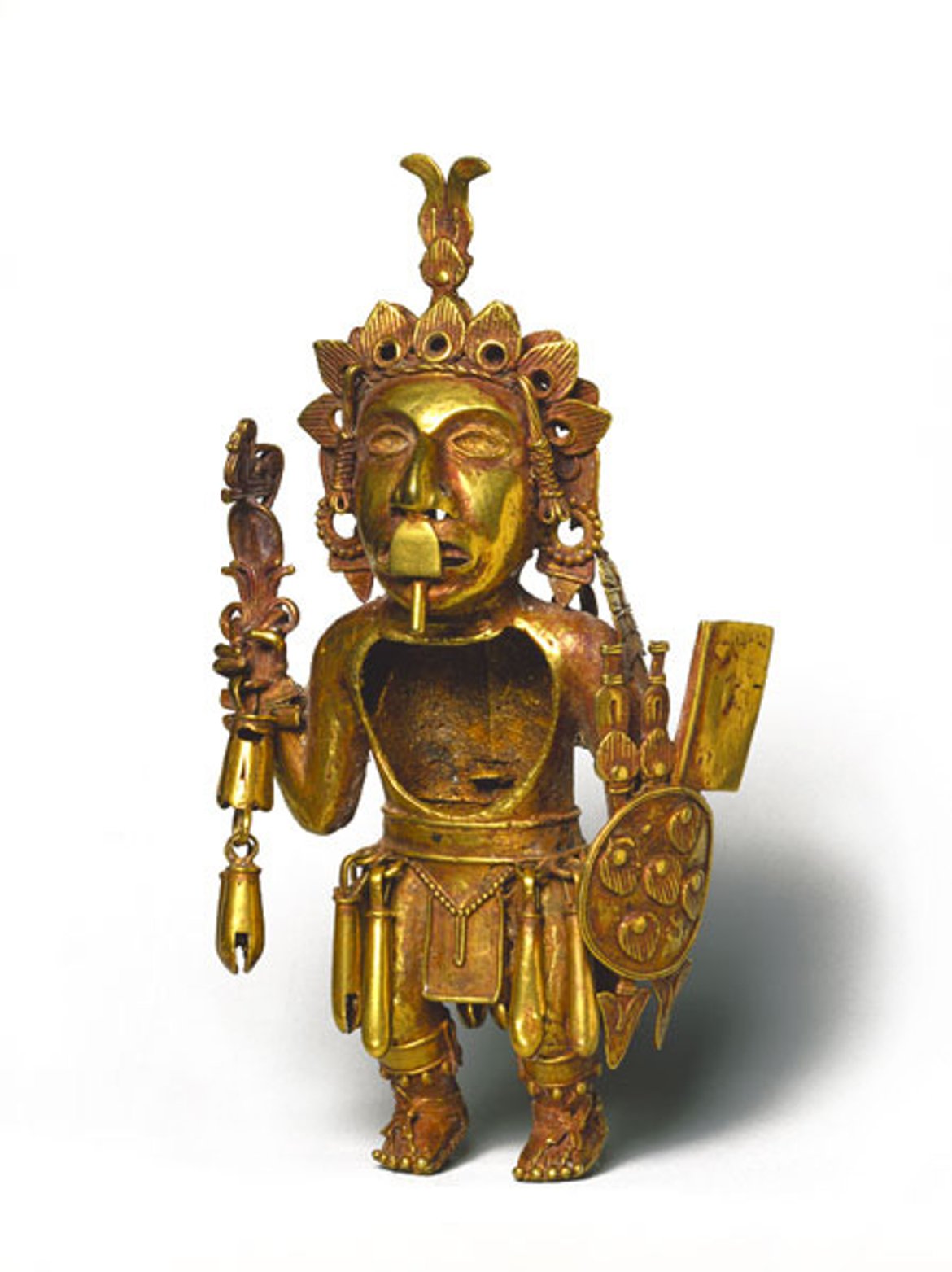The image depicts a small, intricate gold-colored statue that appears to be crafted from a golden material and has notable Native American or Indigenous American artistic elements. The statue features a distinctive face with a prominent nose, from which hangs an ornate oval-shaped metal plate that extends to just beneath the chin. The figure's chest is hollow, revealing what seems to be rusted metal inside. The shoulders and parts of the statue are adorned with a red varnish, adding a vivid accent to its appearance.

On the statue's head, there is an elaborate headdress resembling a bird with wings outstretched to the left and right, embellished with U-shaped and leaf-like details that may represent feathers or leaves with tiny holes. The ears are adorned with large earrings. One hand of the statue holds a complex object that resembles a long staff with two attached bells, possibly a musical instrument.

The other hand grasps a shield that extends past the figure's hip, accompanied by two downward-pointing spears and what might be a rectangular-shaped axe. The statue also wears a belt with dangling gold rods in front of its legs, adding to its ornate attire. Overall, the statue's detailed attire and accessories suggest it is a ceremonial or symbolic piece, representing a rich cultural heritage.